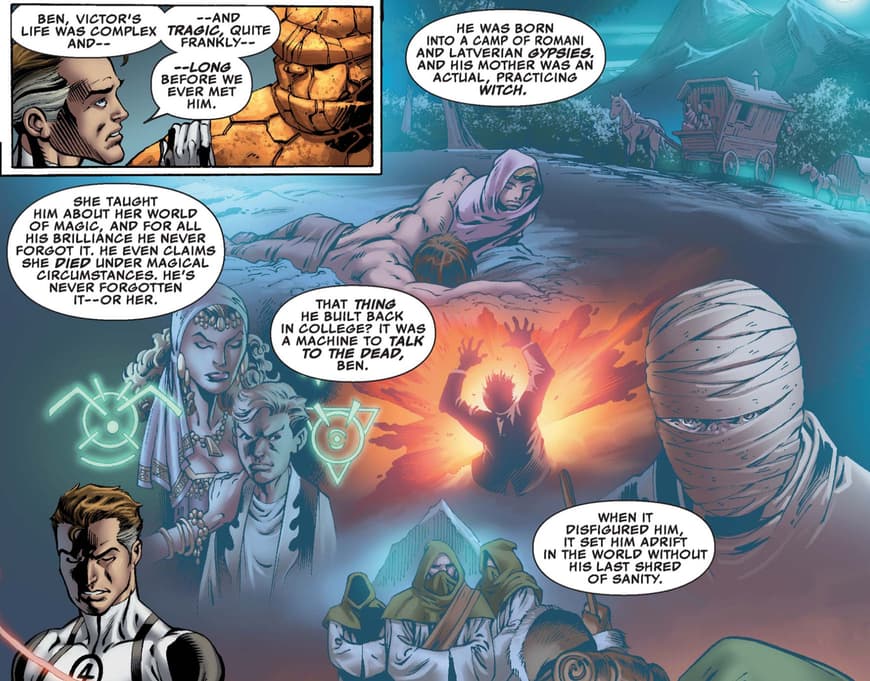This detailed comic book page depicts multiple dynamic scenes and characters. In the top left corner, it features two illustrated characters—one, made of stones, brown in color, and the other, a normal man whose face is visible, engaged in a conversation. The dialogue, contained within white bubbles and written in black capitals, reads, "Ben, Victor's life was complex and tragic, quite frankly, long before we ever met him."

The rest of the page displays a variety of settings and characters, unified by a predominantly blue and purple color theme. One scene showcases a man on the ground next to a horse-drawn chariot, suggesting movement or transition. Another setting features a dramatic explosion with a man being propelled into the air. A mysterious figure, reminiscent of a mummy, appears with his face wrapped in cloth, exposing only his eyes.

Further down, additional characters dressed in robes with face coverings and hoods add to the array of figures, intriguingly placed among symbols glowing in green. The colorful and intricately drawn illustrations offer a vivid storytelling experience, combining elements of action, mystery, and dialogue.